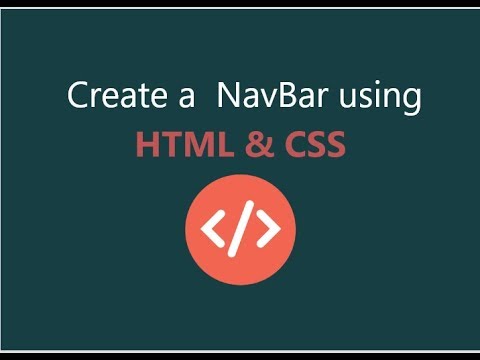This image features a minimalist screenshot set against a clean, solid white background. Dominating the center is a forest green rectangle with a horizontal orientation, significantly extending beyond its vertical height. The green rectangle is framed by a delicate white line, which is further bordered by a thin black line both above and below, creating a subtle yet defined perimeter.

Inside the green rectangle, bold white text is centrally aligned, prominently displaying the phrase "Create a Navbar" followed by a slightly smaller text aligned portion stating, "or navbar using." Directly below this, in bold orange text, are the letters "HTML" and "CSS," all in uppercase, indicating the technologies in use.

Beneath these textual elements lies a large red circle containing white text symbols: a less-than sign, a forward slash, and a greater-than sign, all arranged intuitively to represent the closing tag in HTML code. This visually striking motif underscores the technical theme of the image.